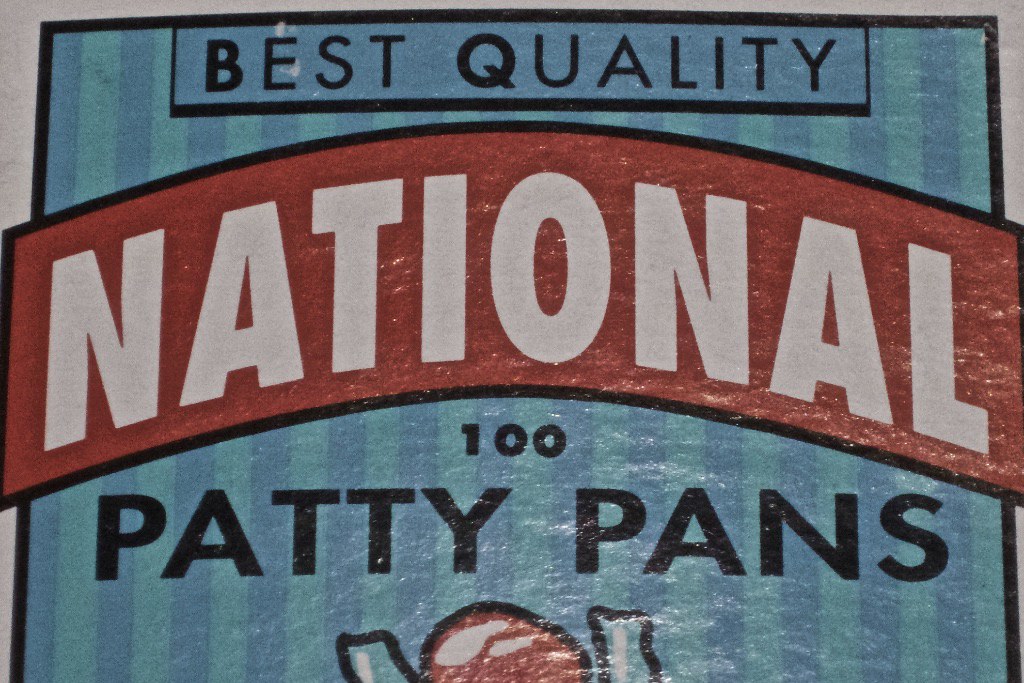The image is a close-up shot of a blue sign featuring vertical light green stripes. At the top of the sign, the words "BEST QUALITY" are printed in black capital letters, with the letters "B" and "Q" distinctly bolded. A red banner cuts across the sign, displaying the word "NATIONAL" in bold, capital letters. Below the banner, the number "100" is prominently featured in bold numerals. Further down, the term "PATTY PANS" appears in capital letters. The bottom section of the sign includes an image, though it is unfortunately cut off and unidentifiable. The sign overall suggests a high standard or premium product related to "patty pans."